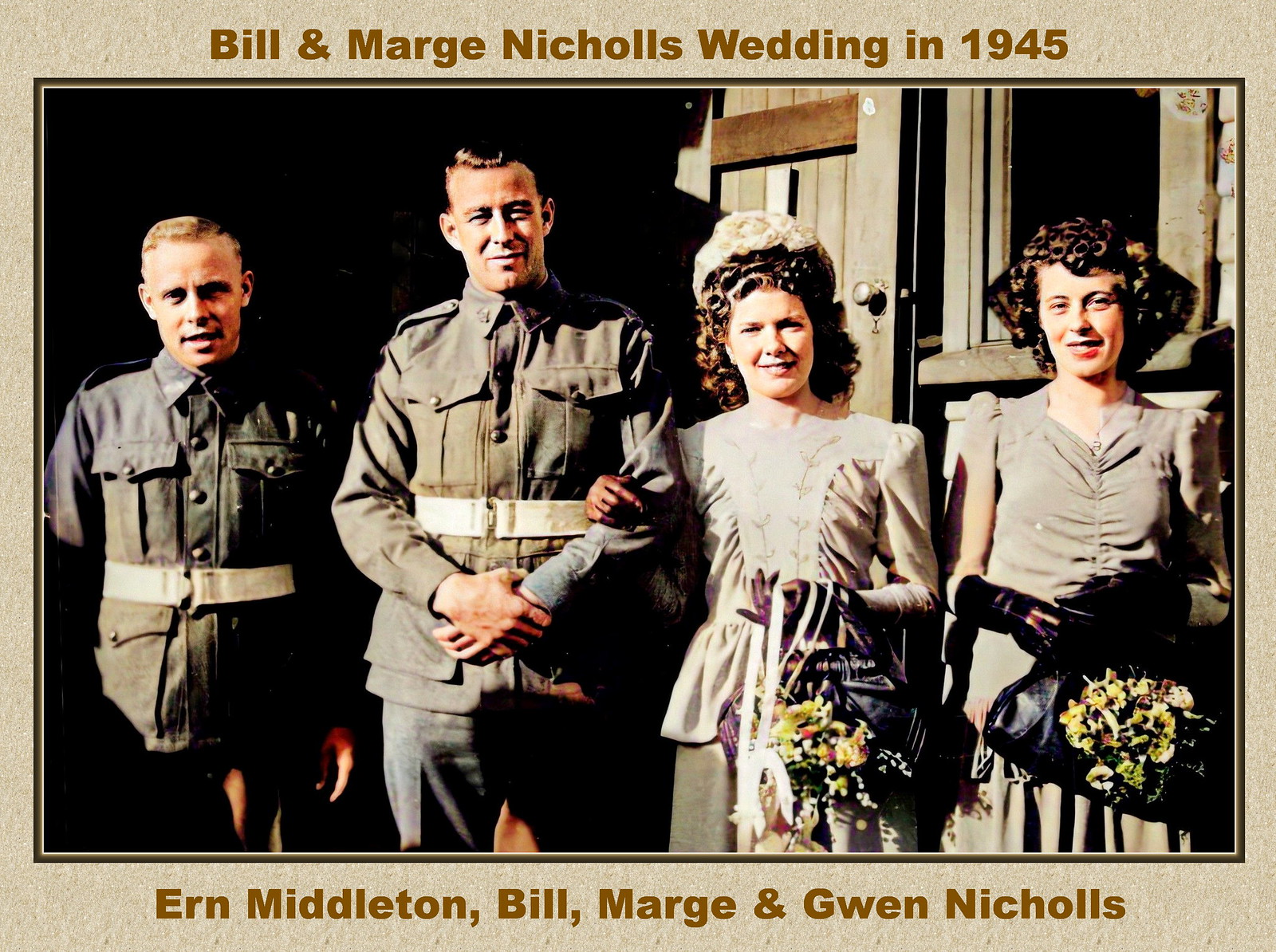This image, likely printed on cardstock with visible individual fibers around the border, shows a color photo from Bill and Marge Nichols' wedding in 1945. The tan or cream-colored card features brown font at the top and bottom, reading "Bill and Marge Nichols Wedding in 1945" and "Earn Middleton, Bill, Marge, and Gwen Nichols." The photo, occupying most of the card, depicts four individuals from left to right. 

On the far left stands a man named Earn Middleton, identifiable by his short blonde hair and dressed in a dark green military uniform. Next to him is Bill Nichols, the groom, slightly taller with short brown hair, also in uniform with his hands clasped together in front. Beside Bill is Marge Nichols, the bride, wearing a white top and skirt, her curly brown hair adorned with a hat. She holds a bouquet of flowers in her left hand, and her right arm is affectionately interlocked with Bill's left arm. To Marge's right is Gwen Nichols, the maid of honor, with short curly brown hair and attired in a light gray dress and black gloves. She carries a purse embellished with flowers in front of her. The formal attire and details, such as bouquets and interlocked arms, emphasize the celebratory moment at the heart of this vintage wedding portrait.